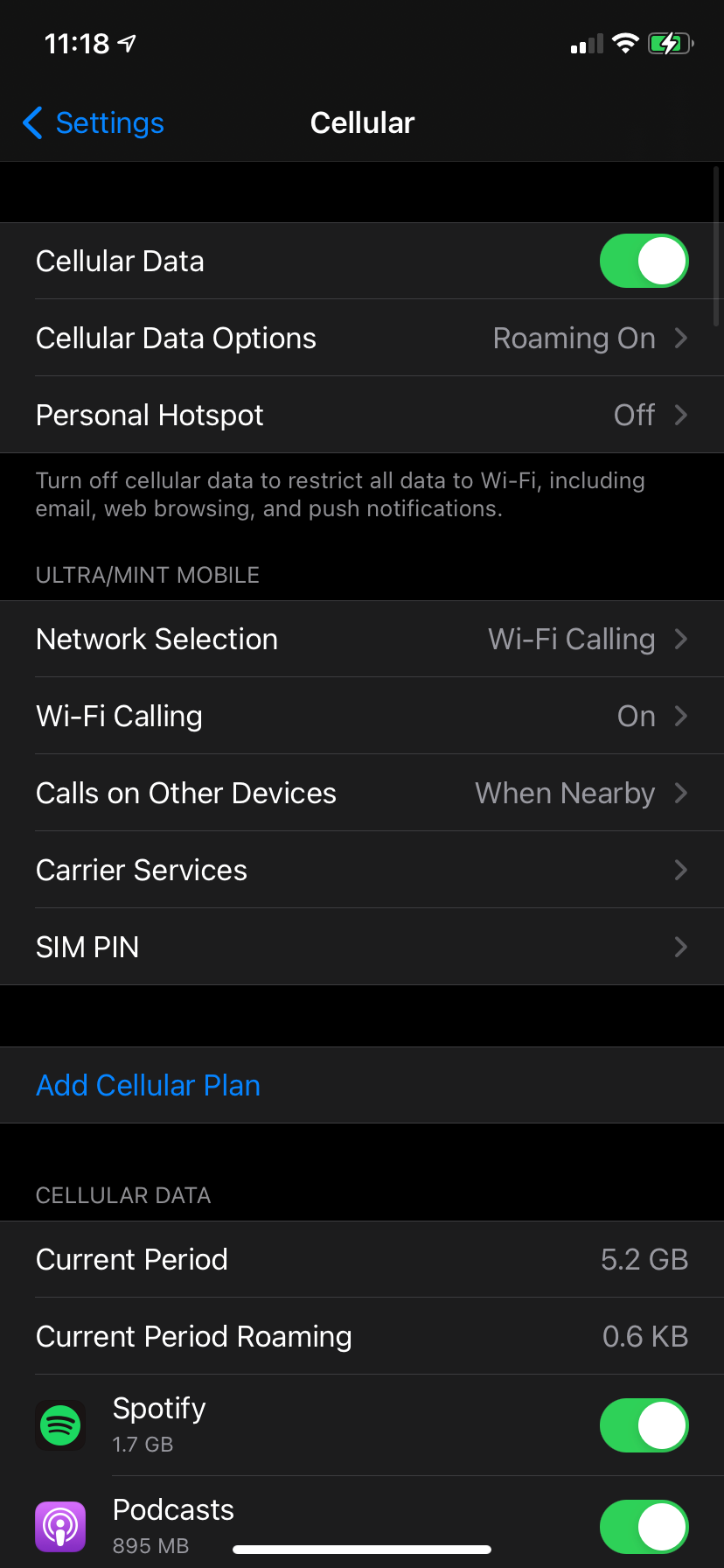Screenshot of an iPhone Cellular Settings Page

In this detailed screenshot of an iPhone's cellular settings, several key details are captured:

- **Top Left Corner**:
  - The time is displayed as 11:18 AM.
  - There is a location toggle icon next to the time.

- **Top Right Corner**:
  - A signal strength indicator shows two out of four bars filled.
  - The Wi-Fi strength indicator displays full bars.
  - A battery icon is present, shown in green, indicating that the iPhone is mostly charged at around 80% and is currently charging.

- **Main Settings Interface**:
  - The current section is "Cellular," as indicated by the title at the top center.
  - To the top-left of the interface, there is a "Settings" label in blue text with a leftward-pointing blue arrow, allowing users to go back to the main settings menu.

- **Options Listed (Top to Bottom)**:
  - **Cellular Data**:
    - Indicated as being toggled on.
  - **Cellular Data Options**:
    - Indicates that roaming is enabled.
  - **Personal Hotspot**:
    - Currently turned off.
  - A text notice below these options: "Turn off cellular data to restrict all data to Wi-Fi including email, web browsing, and push notifications."
  - Further details include carrier information, "Ultra / Mint Mobile."
  - Additional options:
    - Network Selection
    - Wi-Fi Calling
    - Calls on Other Devices
    - Carrier Services
    - SIM PIN
  - **Add Cellular Plan**:
    - Displayed in blue text, indicating it is a clickable option.

- **Data Usage Information**:
  - **Current Period** and **Current Period Roaming** are listed.
  - Below this, there are two apps specified for data usage:
    - **Spotify**
    - **Podcasts**
  - Both apps have their data usage toggles turned on.

This meticulous capture provides a comprehensive view of the current cellular settings and configurations on the iPhone, offering insight into various features and statuses like mobile data, roaming, and personal hotspot settings.